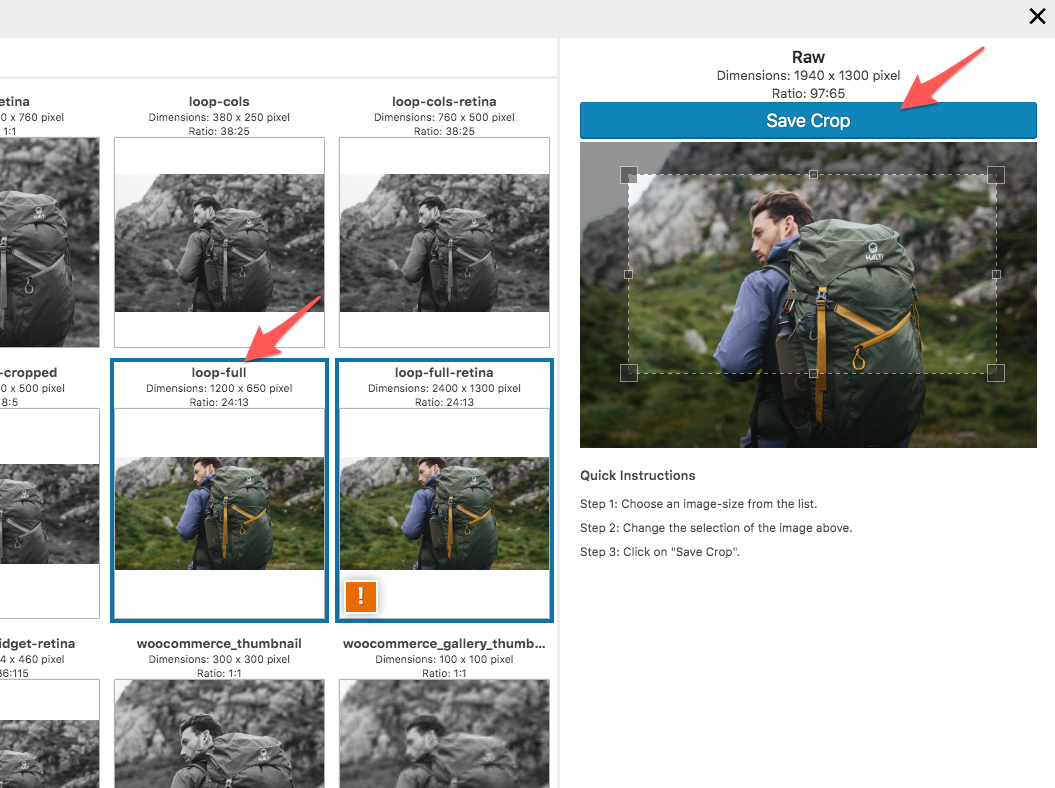The image features a grid of nine smaller pictures of the same person arranged in three rows and three columns, though the entire leftmost column is missing due to the crop, leaving only six visible images. Each of the small pictures is labeled with details such as a name, dimensions, and aspect ratio. On the right-hand side, there is a vertical window marked "Raw," suggesting it displays the selected image in its original form before any edits. When an image is selected from the left, it appears in this "Raw" section on the right. This right-hand section also allows for cropping; red arrow points to a "Save Crop" button at the top of the image. The cropping interface includes lines for resizing and moving the crop frame, allowing the user to adjust the area to be cropped either by shrinking or expanding it to fit their desired selection.